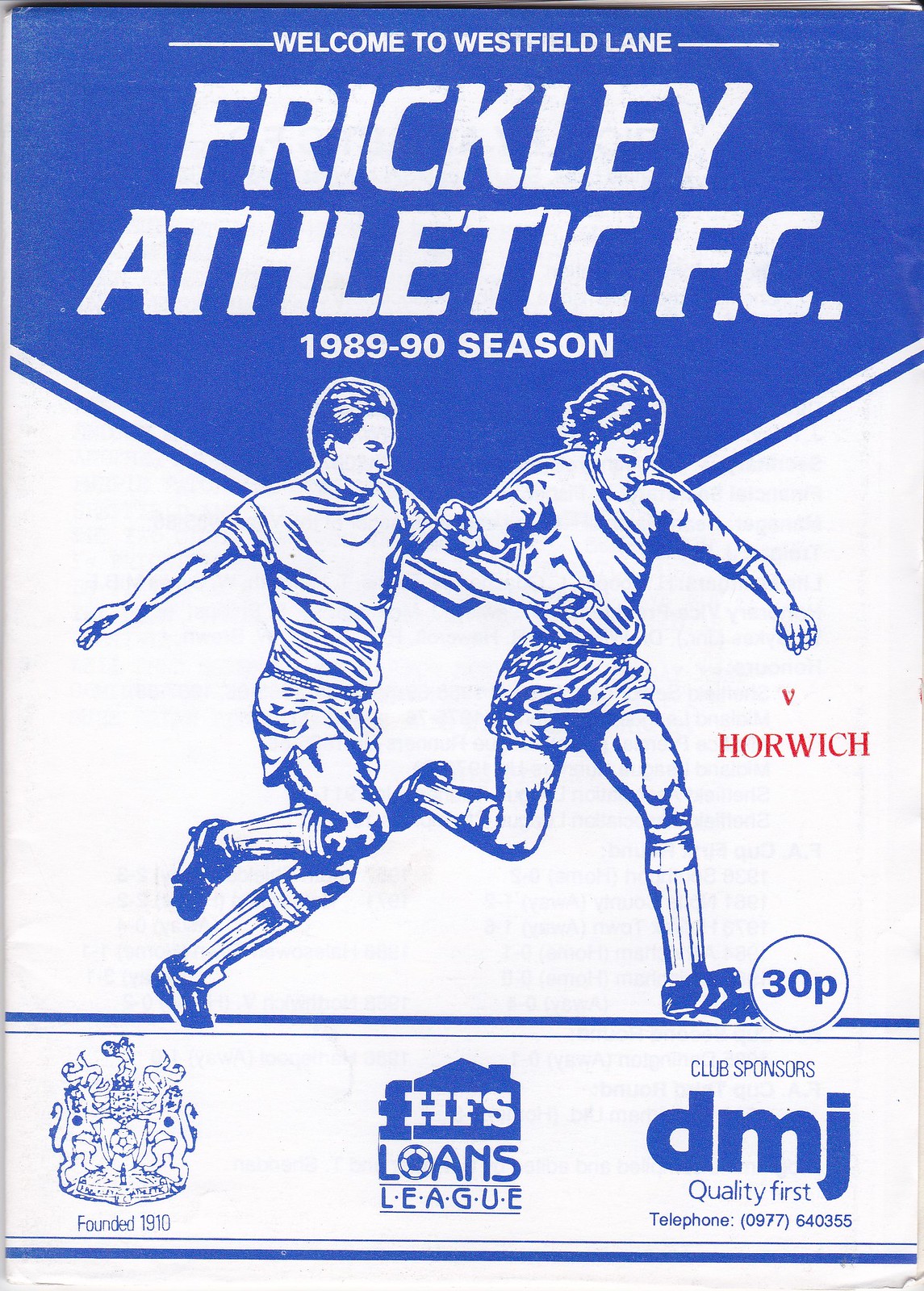The image depicts a vintage soccer program cover from the 1989-1990 season for Frickley Athletic FC, showcasing a blend of white and blue colors. At the very top, there is a V-shaped banner with the text "WELCOME TO WESTFIELD LANE" in small white capital letters, followed by "FRICKLEY ATHLETIC F.C." in larger, bold capital letters. Just below, it reiterates the season: 1989-1990.

Central to the design is a cartoonish sketch of two soccer players engaged in kicking a ball, with one player's foot atop it. The ball features the text "30P," indicating the price of the program. Behind the players, in small red lettering, is an indication of the opposing team, likely "Horwich."

Below the illustrated players, the program features a section divided by a blue band that includes three distinct elements: on the left, the football club's crest with the text "Founded 1910"; in the center, a logo reading "HFS Loans League"; and on the right, an advertisement for the club's sponsors, DMJ, with the slogan "Quality First."

This detailed and nostalgic cover, measuring approximately 4 to 4.5 inches in width and 7 inches in height, serves both as a functional program and a collectible item, encapsulating a piece of Frickley Athletic FC's history.